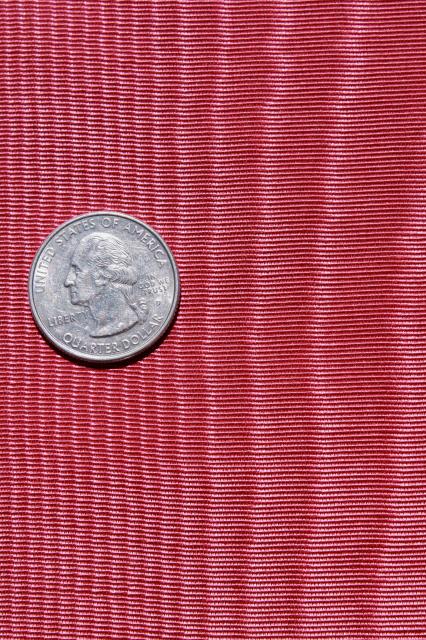A piece of red fabric, resembling corduroy with its characteristic vertical stripes, is folded into several small layers. In the middle of the left-hand side of the fabric lies a well-worn, dull silver quarter. The inscriptions on it, "United States of America," "Quarter Dollar," and "Liberty," are visible, though the date is difficult to discern due to its aged and heavily used condition.